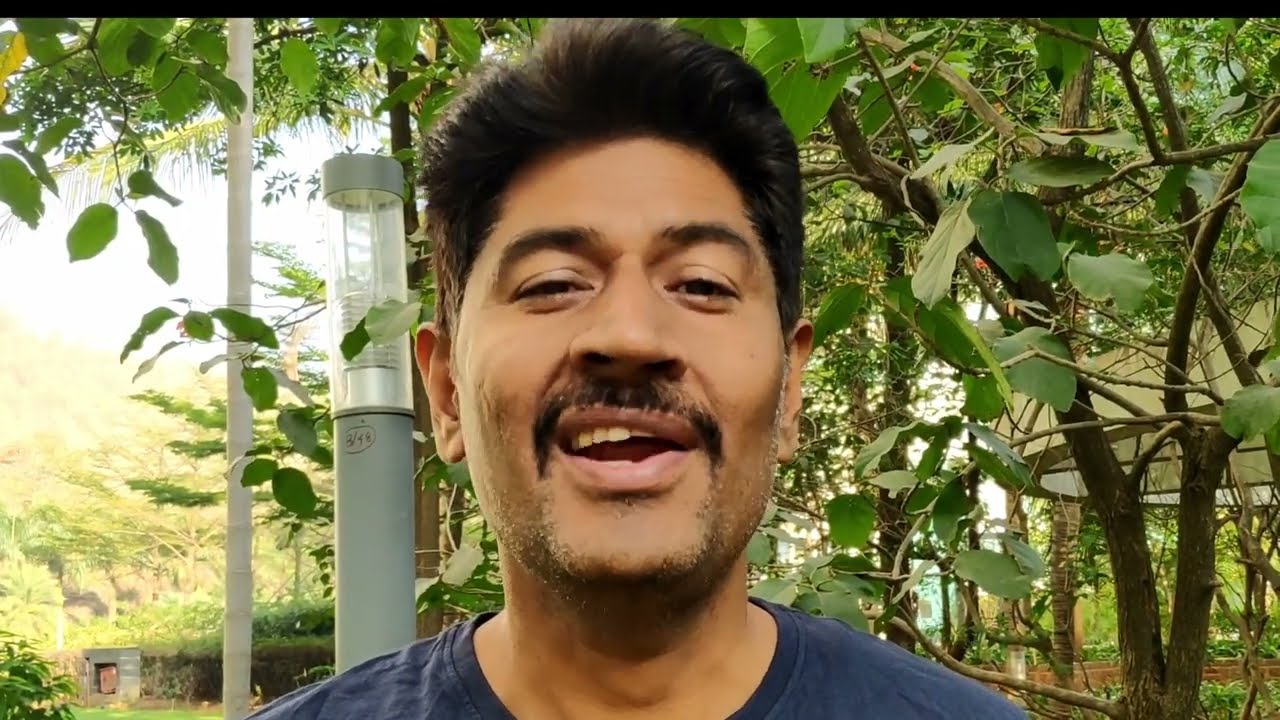The image captures a close-up of a man of likely Arab descent, with dark, slightly fluffy short hair, a mustache, and a goatee. He is wearing a navy-blue shirt and has a half-open mouth with a slight sideways smile, looking directly at the camera possibly in a selfie-style shot. His shoulders, face, and neck are visible in the frame. Behind him, in the distance, is a vast, sunlit landscape featuring a mix of tall, thin trees with green leaves and brown trunks, and some dense greenery suggesting a park-like area rather than a forest. The backdrop also includes a mountainous range and multiple poles: one gray pole with what appears to be a light source at the top, and another taller pole behind it. The bright sunlight illuminates the entire scene, enhancing the vibrancy and detail of the natural elements.